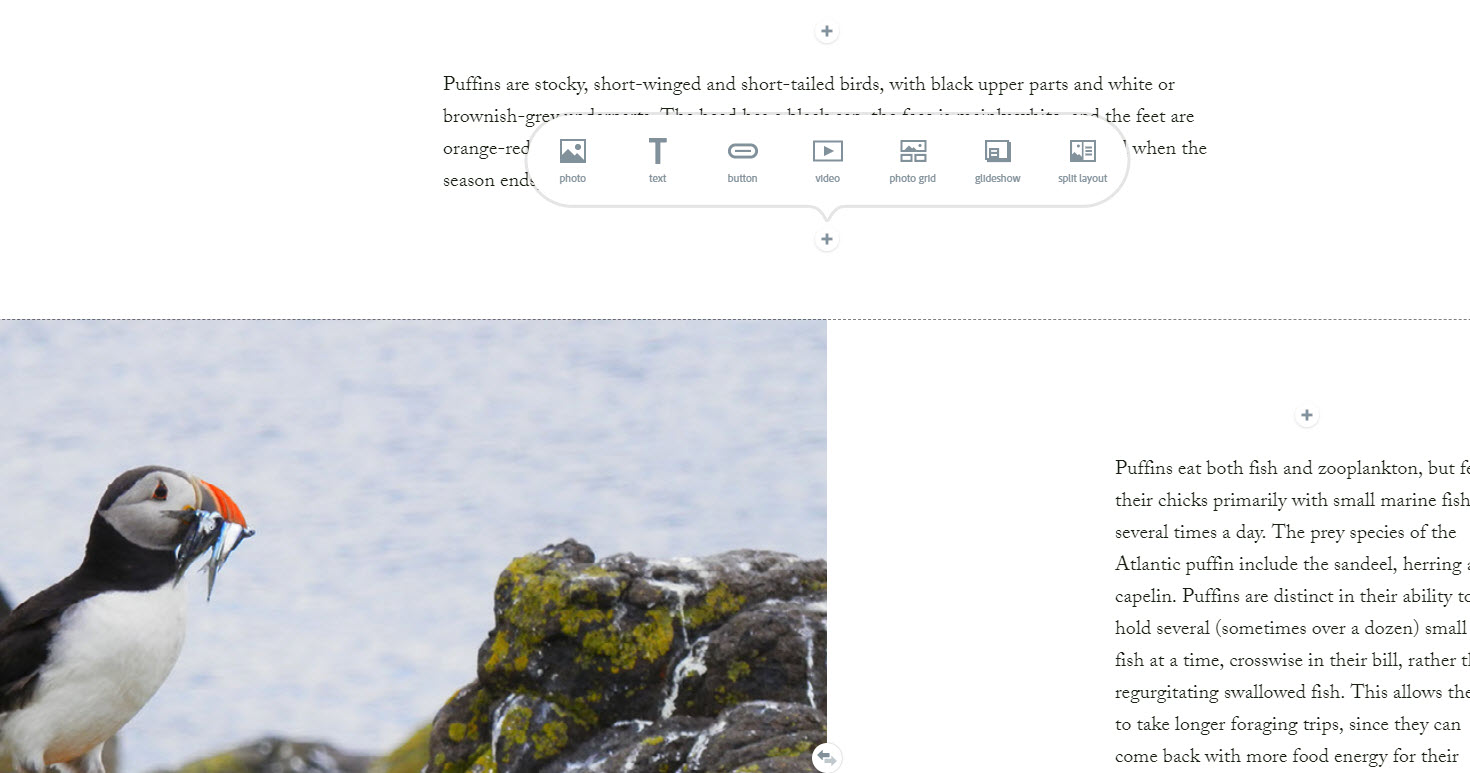The image depicts a webpage under construction, dedicated to puffin information. The layout is wider than it is tall, set against a white background. At the top of the page, there's an incomplete text snippet indicating that puffins are "short, stocky winged and short tailed birds with black upper parts and white or brownish," partially obscured. 

A circular plus icon is positioned above this text, with another plus icon below it. Extending from the bottom plus icon, an oval-shaped interface invites the user to input elements like photos, text, buttons, and more. Below this input area, a gray dotted line spans the entire width of the page.

On the left side, there's a charming image of a puffin holding small fish in its beak, with a watery background and moss-covered rocks in the lower right corner. To the right of this image, a left-justified paragraph provides details about the puffin’s diet, stating that they consume both fish and zooplankton. However, the text is cut off along the right edge, indicating design adjustments in progress. This paragraph further elaborates on the types of fish preferred by different puffin species.

Overall, the webpage is being designed to focus on puffins, particularly highlighting their physical characteristics and dietary habits.